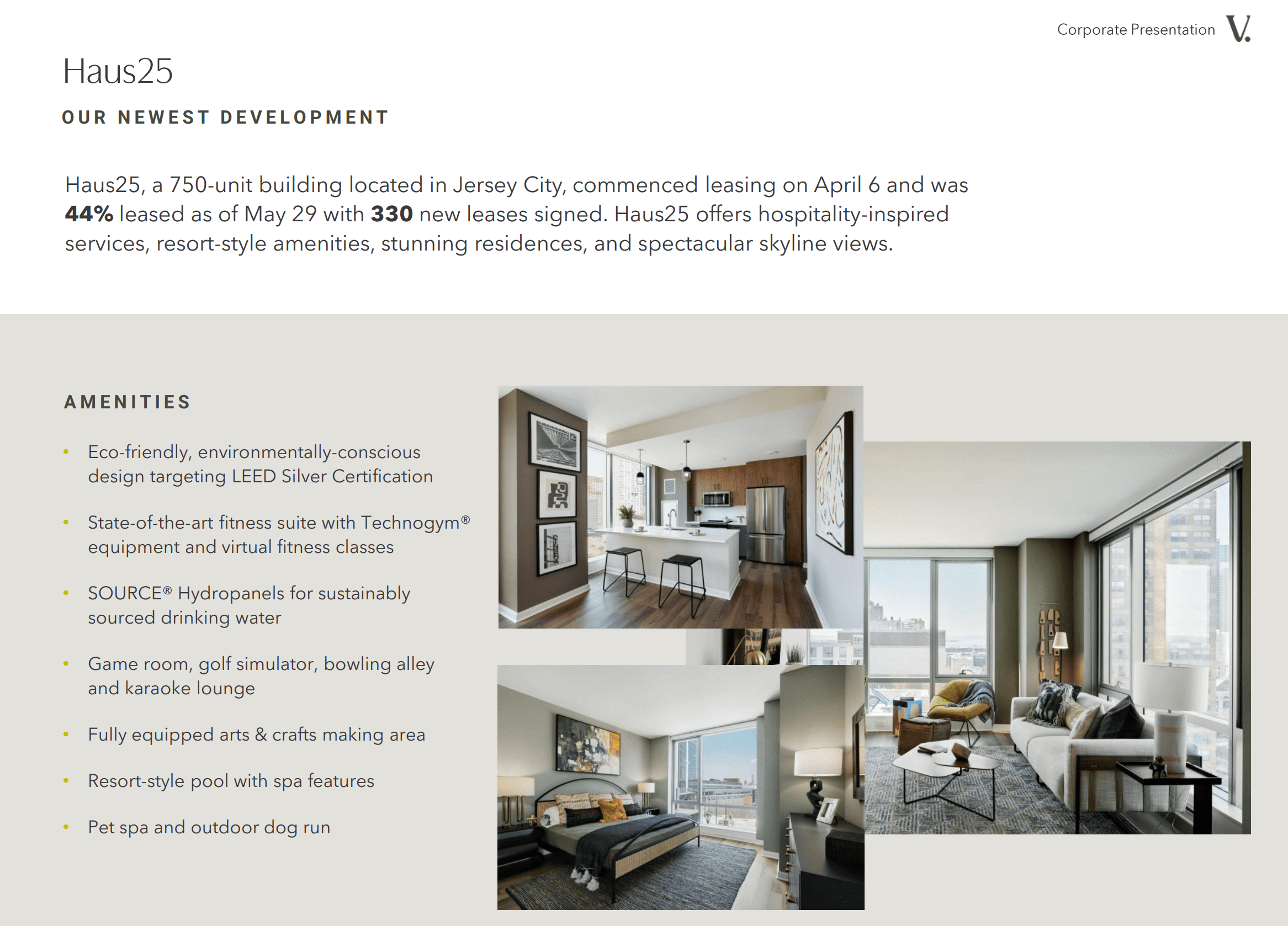**Caption:**

This screenshot showcases a corporate presentation slide for House 25, a newly developed apartment building in Jersey City. The header, "House 25," features a simple white background with black text. In the upper left-hand corner, it reads, "House 25, our newest development," while the upper right-hand corner states, "Corporate Presentation V."

The slide describes House 25 as a 750-unit building that began leasing on April 6th and achieved a 44% leasing rate by May 29th. Below the descriptive text, there is a taupe or beige eggshell-colored rectangle. On the left side of this rectangle, a list of amenities is detailed, including an eco-friendly fitness suite, hydro panels, a game room, an arts and crafts making area, a resort-style pool, and a pet spa. On the right side of the slide, three photographs display the apartment interiors, highlighting the design and features of House 25.